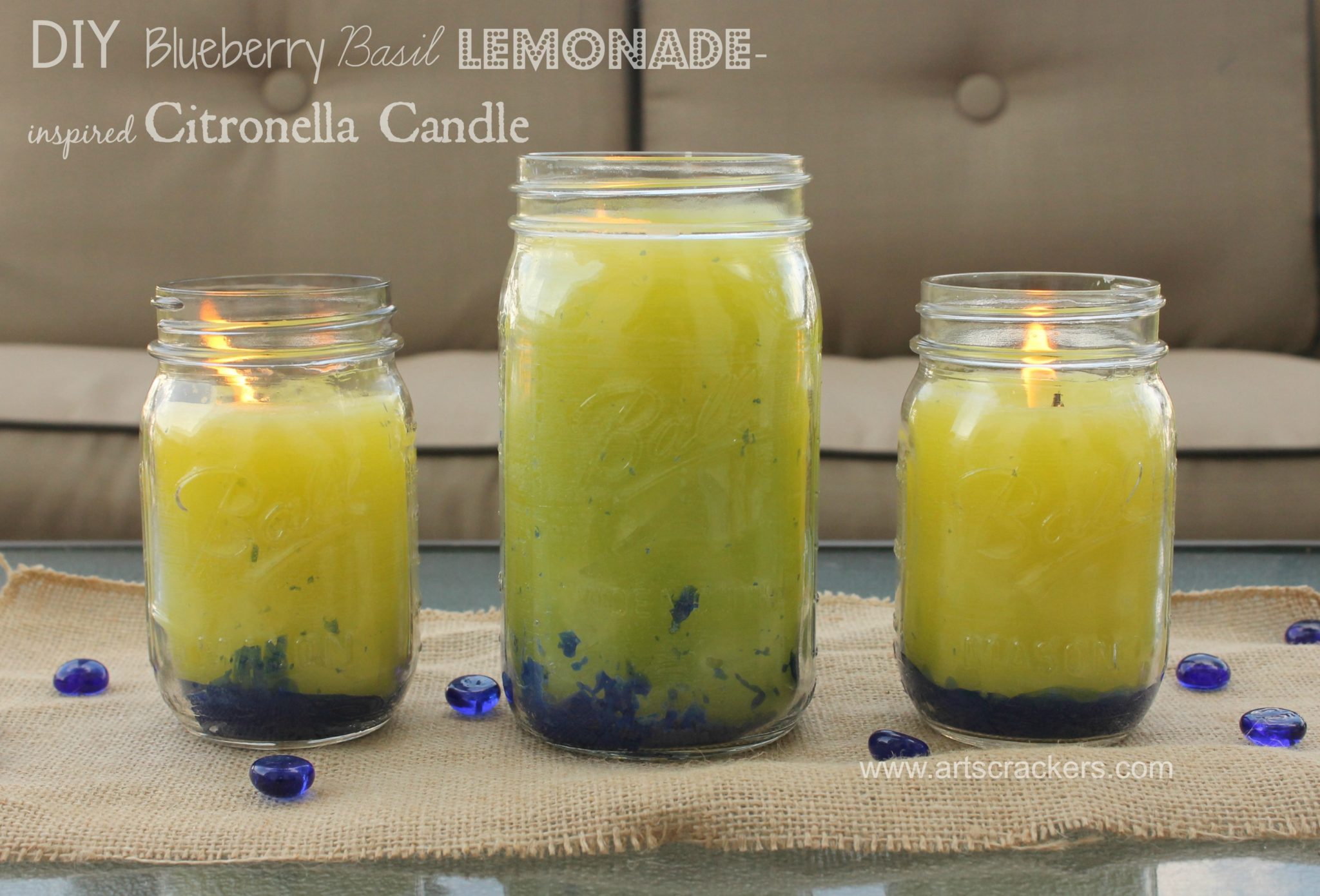In this detailed photograph, three homemade citronella candles are displayed on a glass coffee table in front of a canvas beige sofa. The candles are contained in glass canning jars of varying sizes, with the tallest jar positioned in the center and two smaller jars flanking it on either side. Each candle features a distinct layering of bright blue wax at the bottom and bright yellow wax on top, creating a striking visual contrast.

The jars are placed on a piece of Hessian material, which serves as a rustic base for this arrangement. Scattered around the jars are dark blue and medium blue flat, half-circle glass beads, adding a touch of decorative flair. The lit candles are clearly burning, their flames casting a warm glow over the scene.

In the top left corner of the image, the words "DIY Blueberry Basil Lemonade Inspired Citronella Candle" are prominently displayed. These candles serve as a natural mosquito repellant, combining the fragrant elements of blueberry, basil, and lemonade. This image has a Pinterest-like aesthetic and is likely a feature from the website www.artscrackers.com, showcasing creative and beautifully executed DIY home projects.